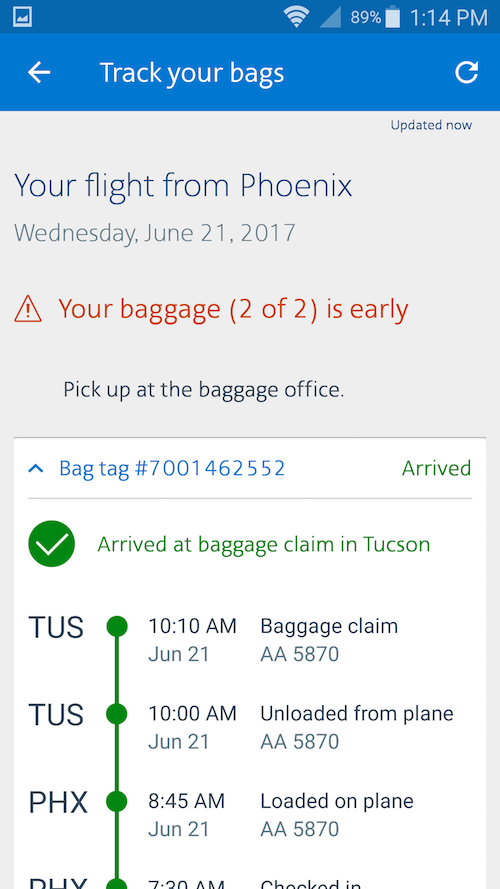The image depicts a smartphone screen displaying a detailed tracking interface for a flight itinerary and baggage check. The screen is predominantly beige and white, with a blue header at the top indicating a flight from Phoenix on June 21, 2017. The app features sections highlighted in green to denote positive updates, and red to signal notifications, which are visually prominent for easy noticeability.

The interface allows users to refresh the tracking status of their bags. According to the screen, the bags associated with a particular bag tag number were checked in at Phoenix, loaded onto the plane, then unloaded at the destination, and finally made available at baggage claim by 10:10 a.m. The various stages of baggage handling are visually represented and time-stamped, indicating an efficient tracking process that took approximately three hours due to time zone differences. The notification in red suggests the bags arrived early, raising the question of whether the bags arrived before the person flying or if they were shipped independently.